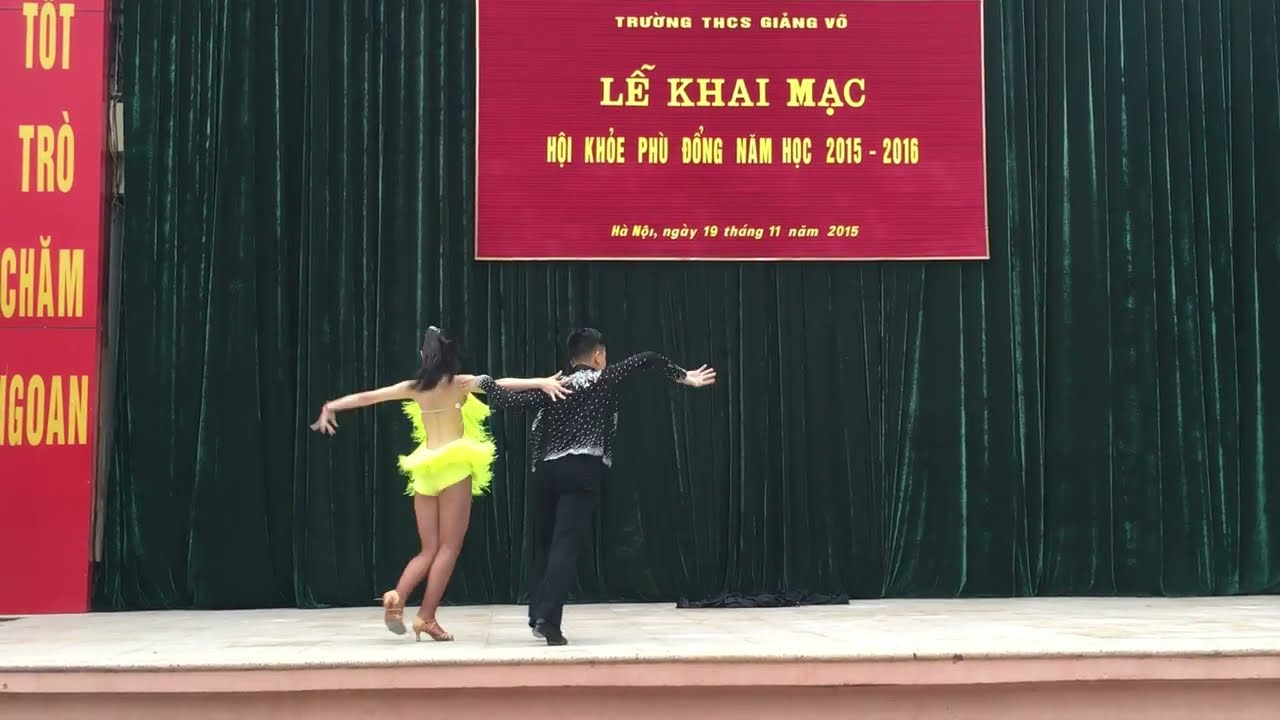In this landscape-oriented color photograph, two young dancers, approximately 10 to 12 years old, are performing on a stage, viewed from the back. The young girl on the left is adorned in a bright yellow, backless, fringe-covered dance costume with a swimsuit-like bottom section and tan, short high heels. Her dark hair is styled in a ponytail, and her arms are outstretched, with her right hand resting on the shoulder of her male dance partner. The boy on the right sports a sparkly black long sleeve shirt with white dots and black pants. Both dancers are poised mid-performance, with the girl's costume's fringe motion captured in the image.

The stage floor is a light beige color, set against a backdrop of rich, black velvet curtains. Prominent red signs with yellow or gold capital lettering in a foreign language are displayed: one hangs at the top middle part of the image, consisting of four lines of text, and another descends from the top to the bottom of the stage on the left side of the photograph. The overall scene is part of an indoor performance, characterized by the vividness of the dancers' attire and the detailed backdrop, emphasizing the photographic realism of the moment.